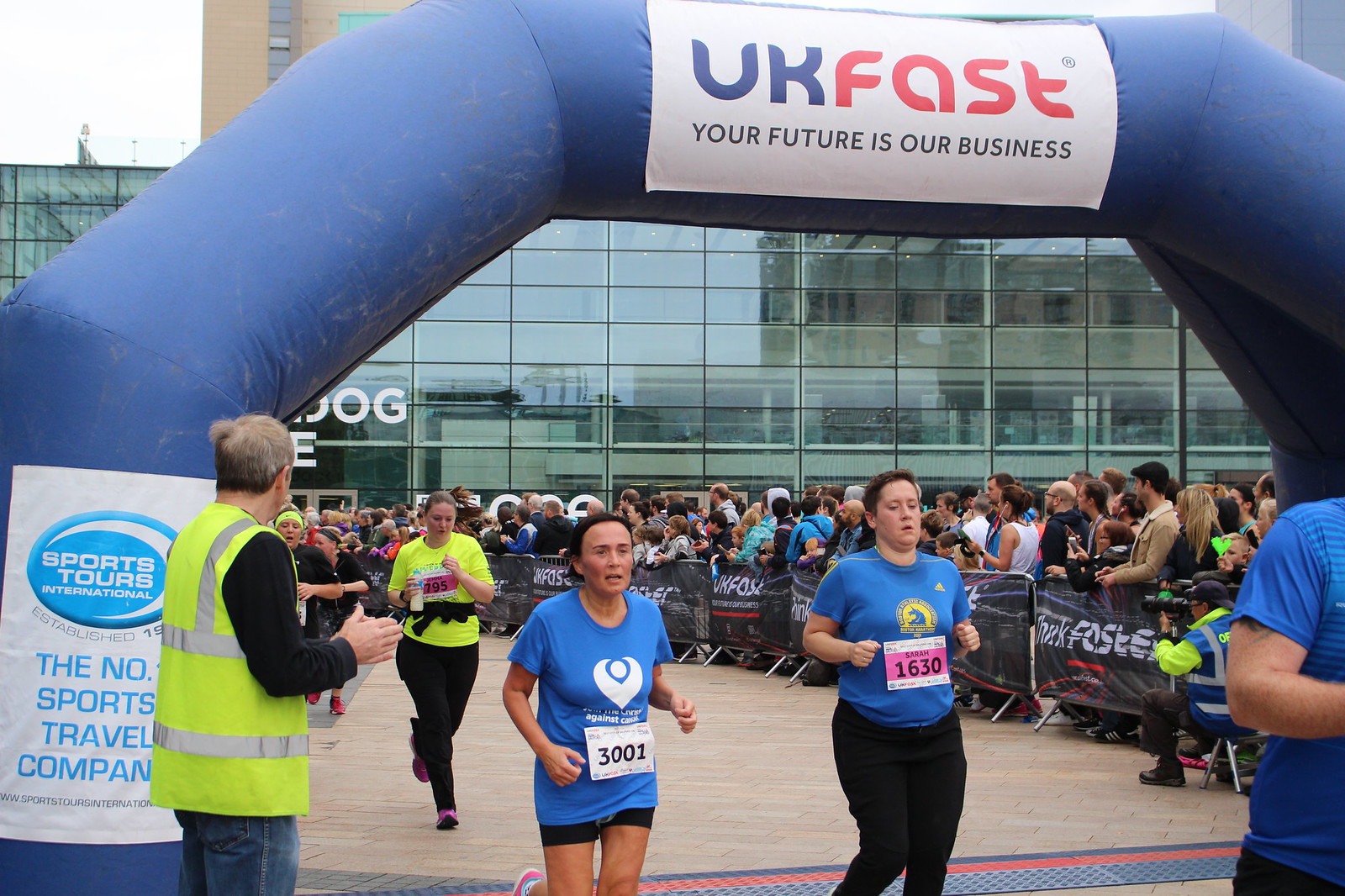In this detailed image description, a race scene unfolds on a concrete surface under a clear, bright midday sky. At the bottom of the image, a large inflatable finish line arch extends upwards and curves overhead, prominently displaying the text "UK Fast" in blue and red, alongside "your future is our business" in black. Additional sponsor text beneath reads "Sports Tours International, the number sports travel company." The scene is bustling with activity as several racers, centered in the image, approach the finish line. 

In focus are three women: the one to the left, wearing a blue shirt and black shorts with the race number 3001, has "Christ Against Cancer" printed on her shirt. Another woman, running slightly behind her, is dressed in a yellow shirt and black pants, while to the right, a runner named Sarah, wearing a blue shirt and black pants, carries the number 1630. A third racer behind them, in black pants, is holding a bottle and wears the number 795. Spectators line the sidelines, forming a large supportive crowd. In the background, beyond the finish line, a building can be seen, adding depth to the outdoor race setting. The scene includes a diverse palette of colors such as white, brown, light green, dark blue, red, black, tan, and lime green, enhancing the vibrancy of the event.